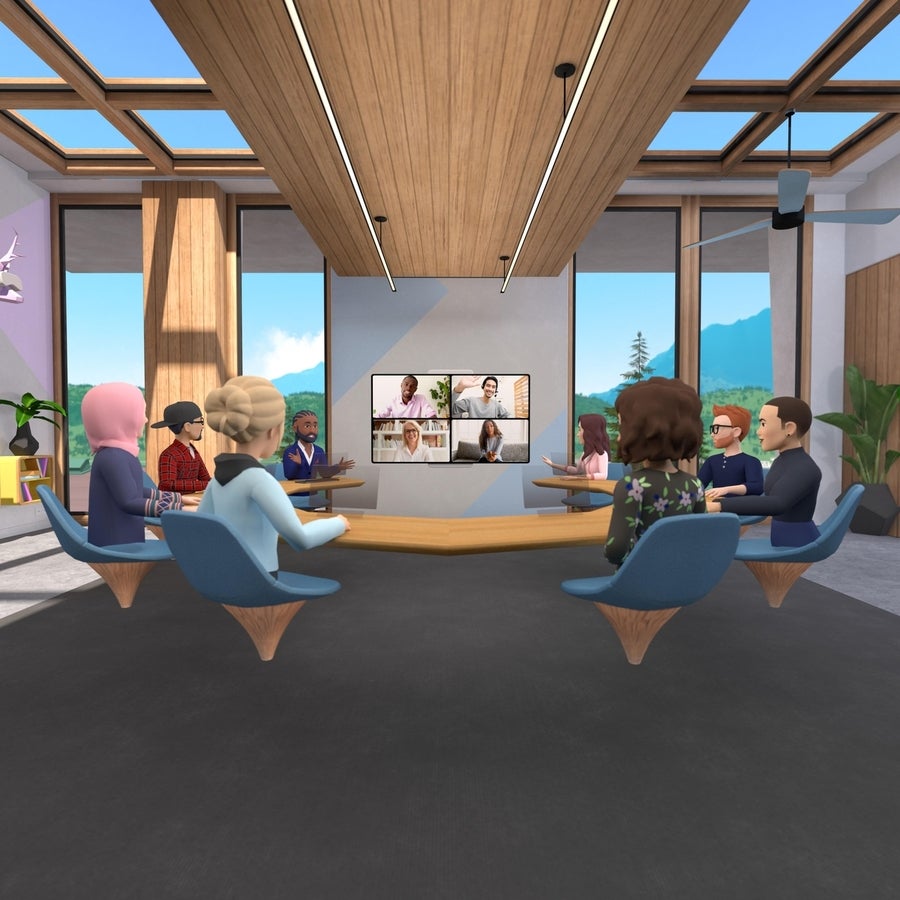The image portrays a business meeting within a conference room styled like a mix of cartoon and video game graphics, reminiscent of Sims characters. Eight digital, model-like characters, dressed in various business attires, are seated around a large, hollow wooden conference table supported on a base that tapers to a small circle on the dark gray floor. They sit on distinctive blue chairs supported similarly, which, along with the table, seem almost to float above the ground. 

The room is spacious and features a brown ceiling with metal rails. A wide television screen at one end of the room is divided into four sections, each displaying a real-life person, contrasting the digital characters around the table. To the left, a yellow bookshelf adds a pop of color to the scene. 

Natural light floods the room through long, narrow floor-to-ceiling windows and skylights, offering a picturesque view of rolling hills, trees, and a blue sky, enhancing the blend of virtual and natural worlds in this unique office setting.